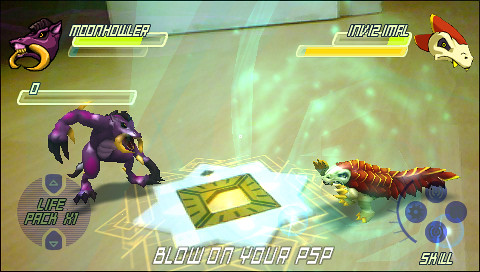This image is a screenshot from an obscure fighting game played on the PlayStation Portable (PSP). The screen showcases two unique characters engaged in combat, reminiscent of games like Street Fighter but featuring monstrous fighters. On the left, a character known as "Moon Howler" appears as a purple warthog or boar with a black mohawk and golden tusks, flaunting a lime green health bar. On the right, another character named "InvisiMole" resembles a small, white dinosaur with a red and yellow head, also equipped with lime green and gold health and shield bars. The interface indicates the player's progress with health and shield bars displayed near the character names, and there is an additional bar below marked '0.' Gameplay icons for moves and attacks are located in circular areas on the left and right sides of the screen. The bottom of the screen prompts players to "Blow on your PSP," suggesting a unique game mechanic activated by blowing air onto the PSP, while additional interface details include "Life Pack X1" and a "Skill" button at the bottom right.